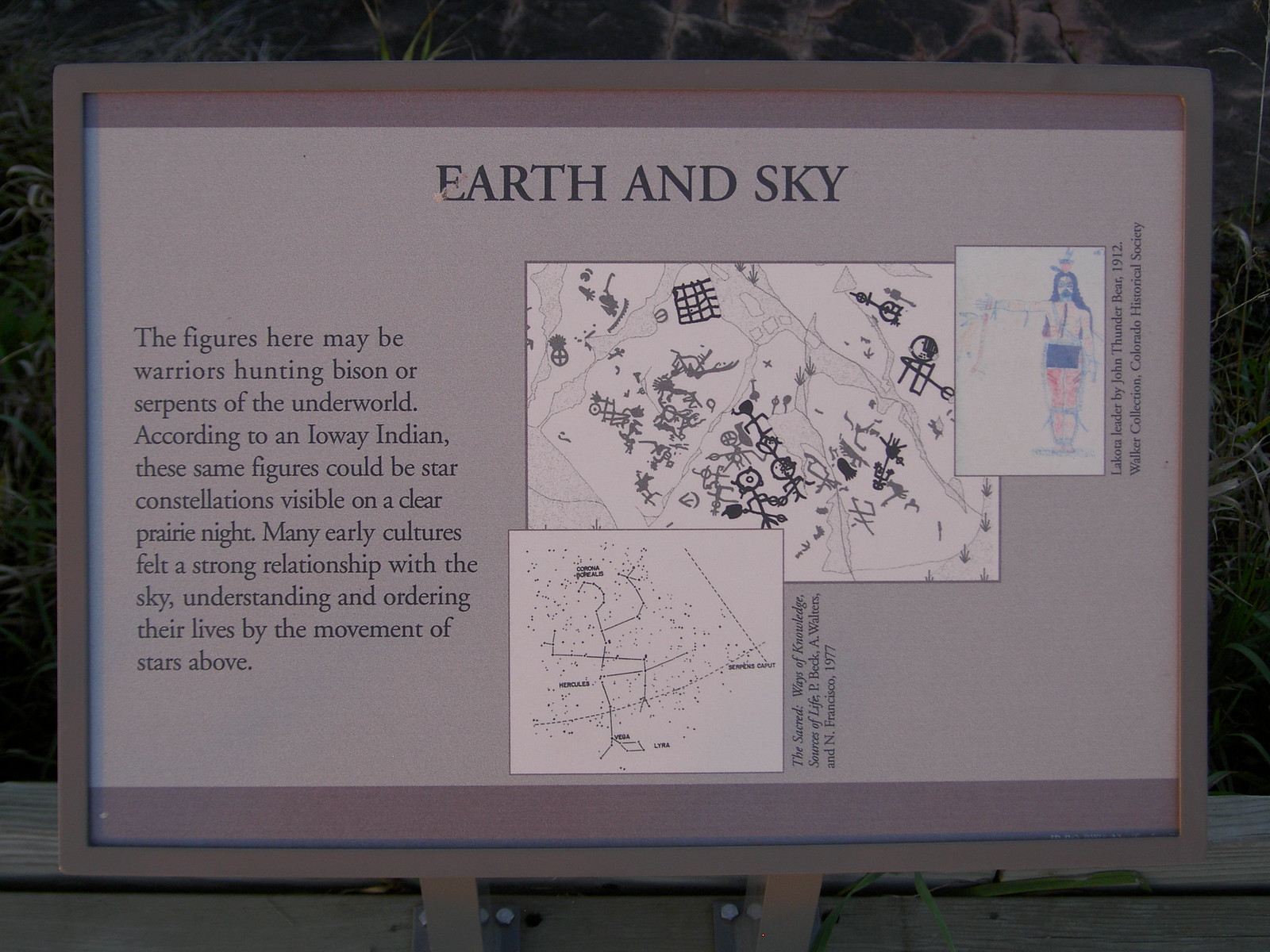The photograph captures an outdoor scene featuring a white-framed informational billboard affixed to a low cement wall, set against a green, grassy or bushy background. The billboard presents historical and cultural insights with the prominent title "Earth and Sky" displayed in black font against a light purple border at the top and bottom of the board. The central focus of the sign includes detailed text and descriptive images. 

On the left side, the text explains that "the figures here may be warriors hunting bison or serpents of the underworld. According to an Iowa Indian, these same figures could be star constellations visible on a clear prairie night." It further elucidates how many early cultures felt a strong relationship with the sky, organizing their lives around the celestial movements.

The billboard features three distinct charts or illustrations. One image, situated at the bottom, depicts star constellations in black on a white background. Another drawing showcases black stick figures equipped with spears, nets, and pitchforks. Among them is a colored depiction of a man with blue hair and a decorative skirt, with his legs represented in red. An additional photograph on the right, containing some color, possibly illustrates a bare-chested gentleman, adding to the eclectic mix of representations. The detailed narrative and visual elements combine to create a thorough educational exhibit on the interplay between ancient cultures, their myths, and their astronomical observations.